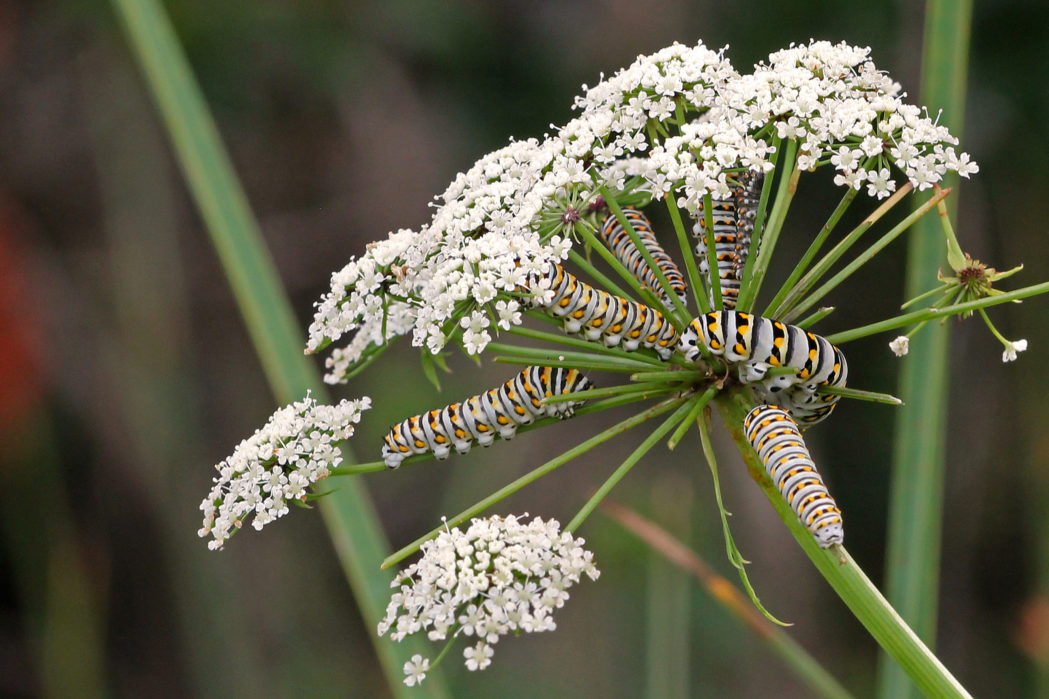The image is a detailed, close-up photograph of a flowering plant set against a blurry, gray-green background, suggesting it was taken either in a garden or the wilderness. The plant features a prominent green stem extending down to the right corner, from which thin branches with clusters of small white flowers sprout in multiple directions. Interspersed among the green parts of the plant are several white caterpillars adorned with distinctive black and yellow stripes. These caterpillars are actively feeding on the plant, with some sections of the branches appearing damaged or partially eaten. Bright red and orange elements—possibly additional flowers—are visible at the perimeter, enhancing the vibrant, natural scene.